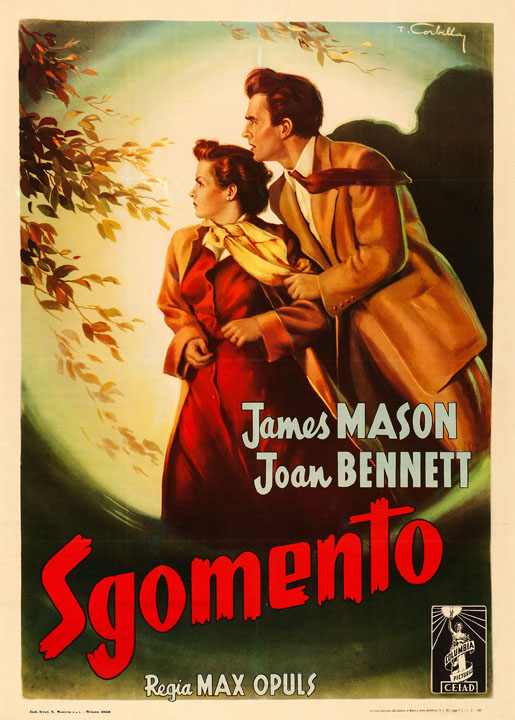The image is an old movie poster featuring an illustration of a man and a woman. The man, with brown hair styled in a pompadour, is dressed in a caramel-colored suit, a red tie, and a white shirt. He is holding the woman by the arm. She has medium red curly hair and is dressed in a red gown with a brown caramel-colored coat and a yellow scarf. Both characters are looking to the left with expressions of curiosity and fear. 

The background showcases a large white moon, casting shadows of the couple. On the upper left, green and red leaves are depicted, adding to the scene. The poster has a beige-colored border with black text in the lower corners, which is too small to read clearly.

Centrally, the names "James Mason" and "Joan Bennett" are written in pale blue letters. The movie title "Sugomento" is prominently highlighted in red at the bottom, with "Regia Max Opuls" written below it in white. A logo featuring the Statue of Liberty is positioned at the lower right corner. The artist's signature appears at the top right in white ink, adding a final touch to this stylized vintage movie poster.